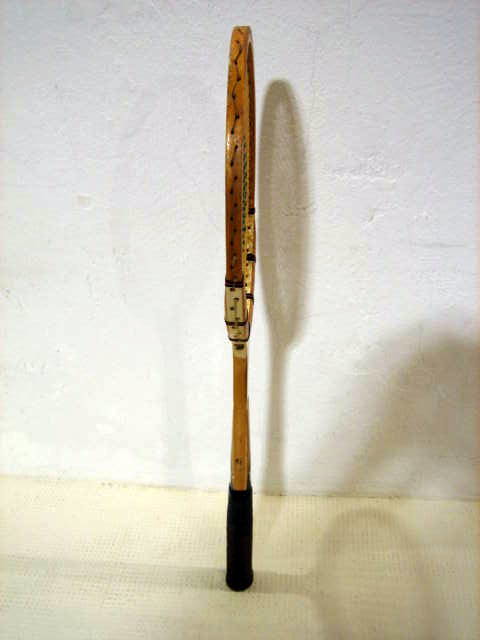This photograph captures a vintage wooden tennis racquet standing upright on its handle against a white concrete wall. The racquet, positioned vertically and viewed from the side, showcases its wooden frame with visible wood grain. The oval head of the racquet features strings threaded through clearly seen holes along its edges. The bottom portion of the frame is detailed with a black line encircling the racquet, transitioning to white and continuing down to a light brown wooden handle wrapped in a black rubber grip. The ground beneath the racquet appears textured, possibly light tan carpeting, casting a shadow against the white wall and the ground itself. The scene is framed to highlight the racquet's antique craftsmanship and its solitary stance in a minimalist setting.